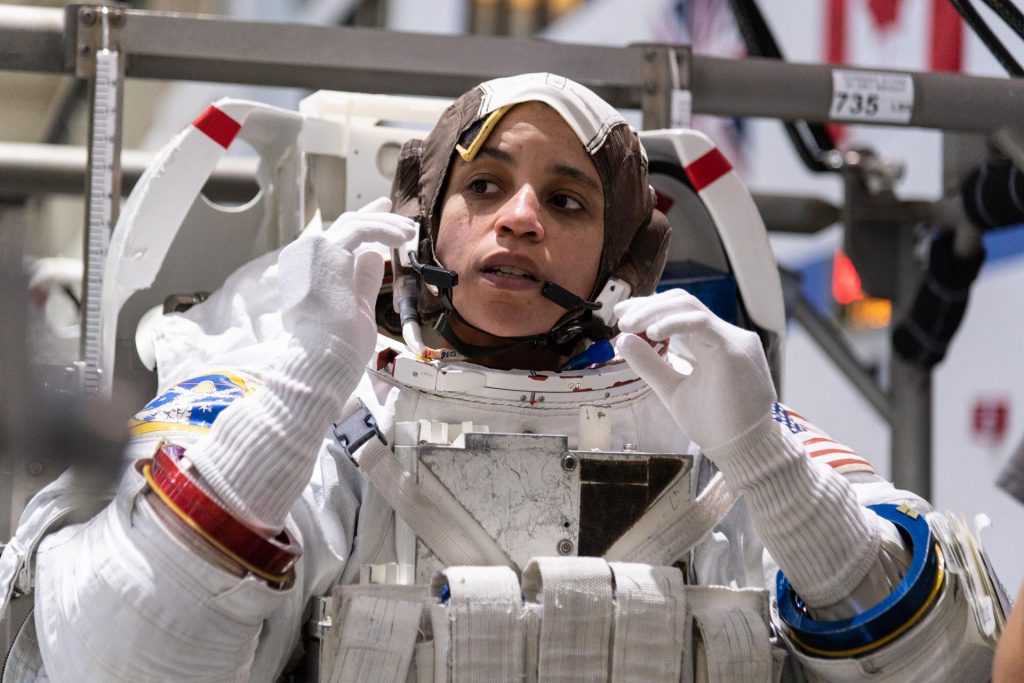This detailed photograph captures a female astronaut in the process of putting on her spacesuit. She is seated in a white chair with red-lined handles on both sides. The astronaut is dressed in a traditional NASA spacesuit, characterized by white fabric and featuring white gloves on her hands. Displayed prominently on her left shoulder is the American flag, while her right shoulder bears a distinct NASA insignia. Straps are visible across her chest, and a backpack or equipment is attached to her back, peeking over her head. Her face, framed by a cloth hood that covers her hair, is clearly visible; she has dark skin and dark mauve lips. Positioned on the side of her head is a device resembling a microphone. In the background, industrial elements such as metal bars, framing, and other equipment are visible, along with the numbers "735" on one of the metal bars. The photograph captures her facing the camera, though her eyes are directed slightly to the side.